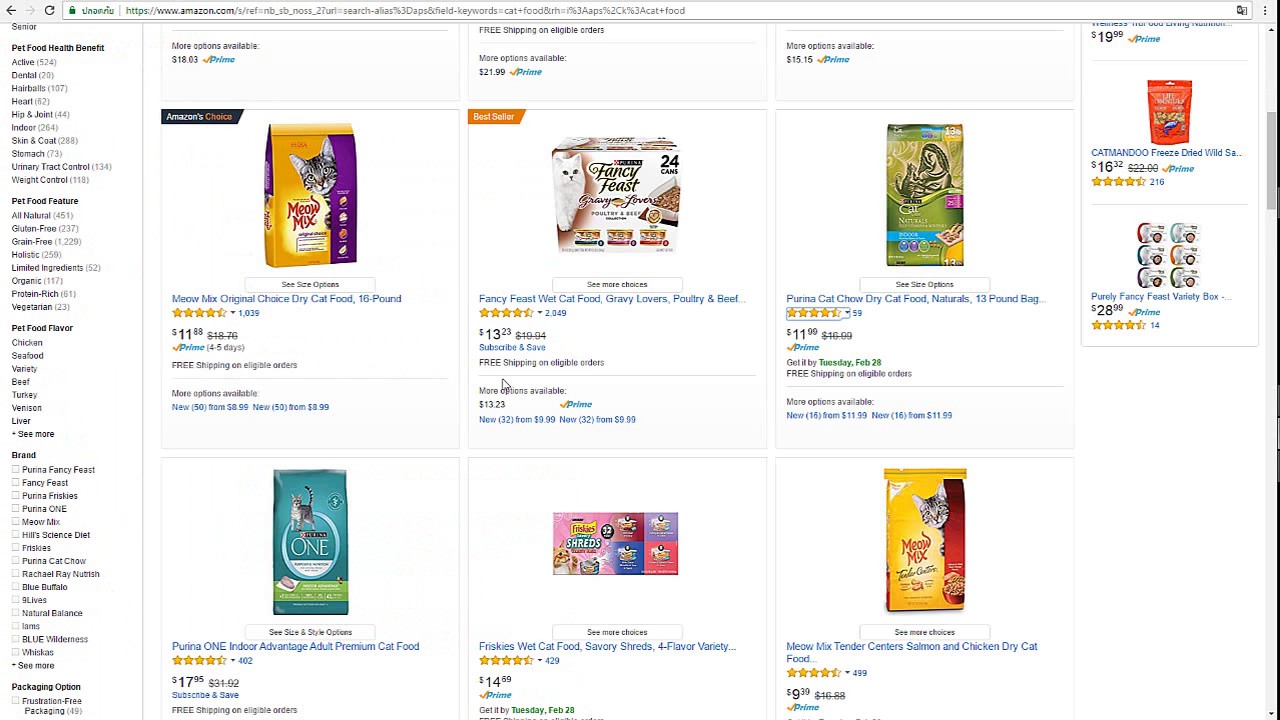The webpage screenshot displays the Amazon.com website, identifiable from the URL in the address bar which includes a string of additional characters. The layout consists of a sidebar on the left and the main section showcasing various cat food products. The top product is labeled "Amazon Choice Meow Mix Original Choice Dry Cat Food, 10 lbs," priced around $11.88, though the exact price is somewhat blurry. It includes the Prime 4-5 days shipping option with free delivery on eligible orders. 

The second product, marked as a "Best Seller," is the "Fancy Feast Wet Cat Food, Gravy Lovers, Poultry & Beef," listed at $13.23 with a subscribe and save option plus free shipping on eligible orders. 

The third listing features "Purina Cat Chow Naturals, Dry Cat Food, 13 lbs. bag," priced at $11.99 with Prime eligibility, promising delivery by Tuesday, February 28th, and including free shipping on eligible orders.

The final product on the bottom left is labeled "Purina One Tender Selects Blend Adult Dry Cat Food," although pricing and specific details are not clearly discernible due to image blurriness.